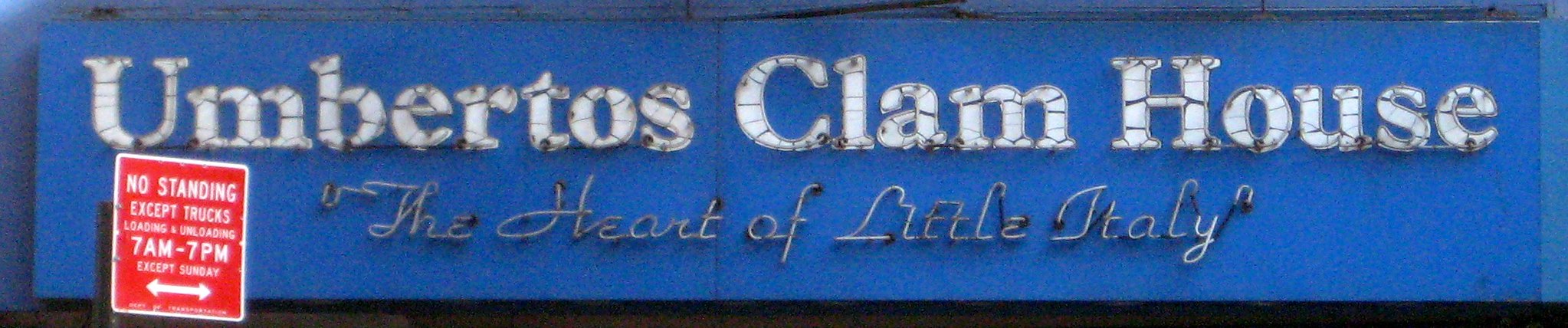The image depicts the blue, rectangular signage of Umberto's Clam House, a restaurant situated in the heart of Little Italy. The sign, which measures approximately 10 inches long by 2 inches wide, is adorned with white bold lettering that reads "Umberto's Clam House," and underneath in white cursive, "the heart of Little Italy." The sign is likely capable of lighting up, though it is currently unlit, suggesting it was photographed during the daytime. The restaurant itself appears to be associated with either a blue or white exterior, reflecting the color of the sign. Additionally, to the bottom left of the main sign, there is a smaller red sign that states, "No standing except trucks. Loading and unloading 7 a.m to 7 p.m except Sundays." This comprehensive view encapsulates the essence and details of the restaurant's presence in Little Italy.